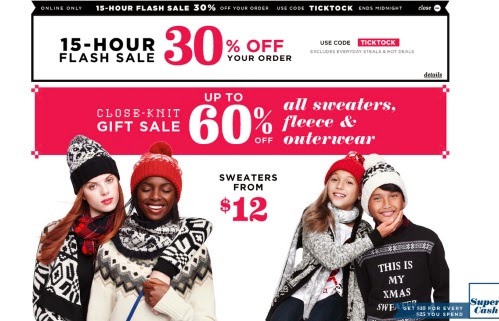**Caption:**

This screenshot showcases a sale promotion with a detailed layout. 

At the top, there is a black border with white lettering on the left side. In small lettering, it reads "ONLINE ONLY," followed by a bold white text stating "15-HOUR FLASH SALE 30% OFF YOUR ORDER." Beside it, in small white lettering, it mentions "USE CODE" and in bold white, "TIKTOK." The offer ends at midnight, as indicated by the small print.

Below this, the background is white with a black border on the left, bottom, and right sides. Centered to the left, bold black text reads "15-HOUR FLASH SALE," with "30% OFF YOUR ORDER" beneath it in smaller bold black text. To the right, in black text, it instructs to "USE CODE," followed by a red rectangle with white text inside that says "TIKTOK." Additionally, black text mentions "INCLUDES EVERYDAY STEALS AND HOT DEALS," and in the bottom right corner, bold black text reads "DETAILS."

Further down, a red rectangle with centered white text announces "UP TO 60% OFF." To its left, in white text, it states "CLOTHES **&** GIFT SALE," and to the right, "ALL SWEATERS, FLEECE & OUTERWEAR."

Below this section, the background turns white, and in the center, black text reads "SWEATERS" with a large red "$12" beneath it. To the left, there's an image of a white girl with red hair wearing a black and white jacket, her arm around an African-American woman. The woman is smiling with her eyes closed and wearing an orange garment with a white and black hoodie or sweater.

On the right side, two young kids are shown. The girl on the left has a red garment, a gray sweater and a white shirt, while the boy on the right is wearing a white, gray, and black outfit along with a black and white shirt.

In the bottom right corner, there's a blue tab with white text that reads, "GET $45 FOR EVERY $25 YOU SPEND."